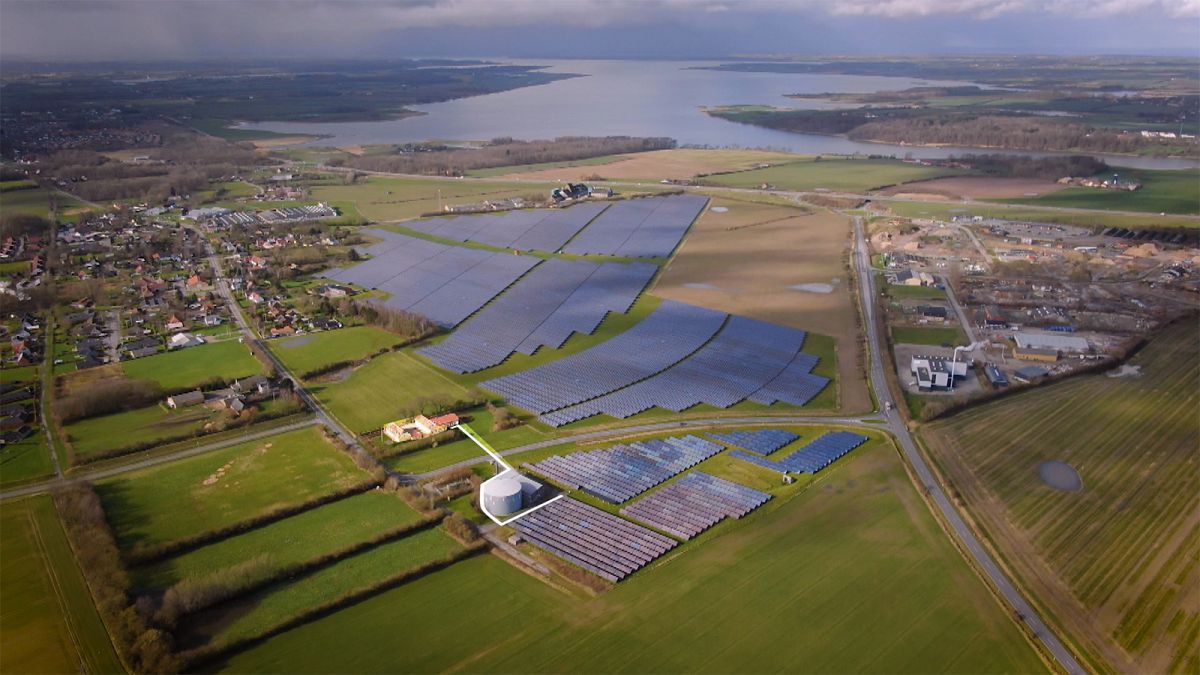This aerial photograph captures a vast rural landscape primarily composed of expansive green fields. Dominating the center of the image is an extensive array of neatly arranged blue and purple solar panels, which occupy a significant portion of the land. Adjacent to the solar farm, on the right side, there is a large white silo connected by white pipes to a substantial white building, suggestive of industrial or agricultural storage facilities.

To the left side of the solar panels, closer to the upper left corner of the image, lies a small, densely packed town with multiple houses and large gray asphalt roads crisscrossing between them. There is a noticeable section of brown farmland with small puddles and lakes directly next to the solar farm, indicating active agricultural use.

Further left, towards the middle center of the image, is a triangular area that appears to be a commercial zone with buildings under construction or existing commercial structures, adding to the landscape's diversity. In the background, beyond the solar farm, lies a large glittering lake with clear blue water under a sky filled with gray clouds illuminated by sunlight. The horizon is visible beyond the lake, emphasizing the expanse and blending the natural and developed elements within the scene.